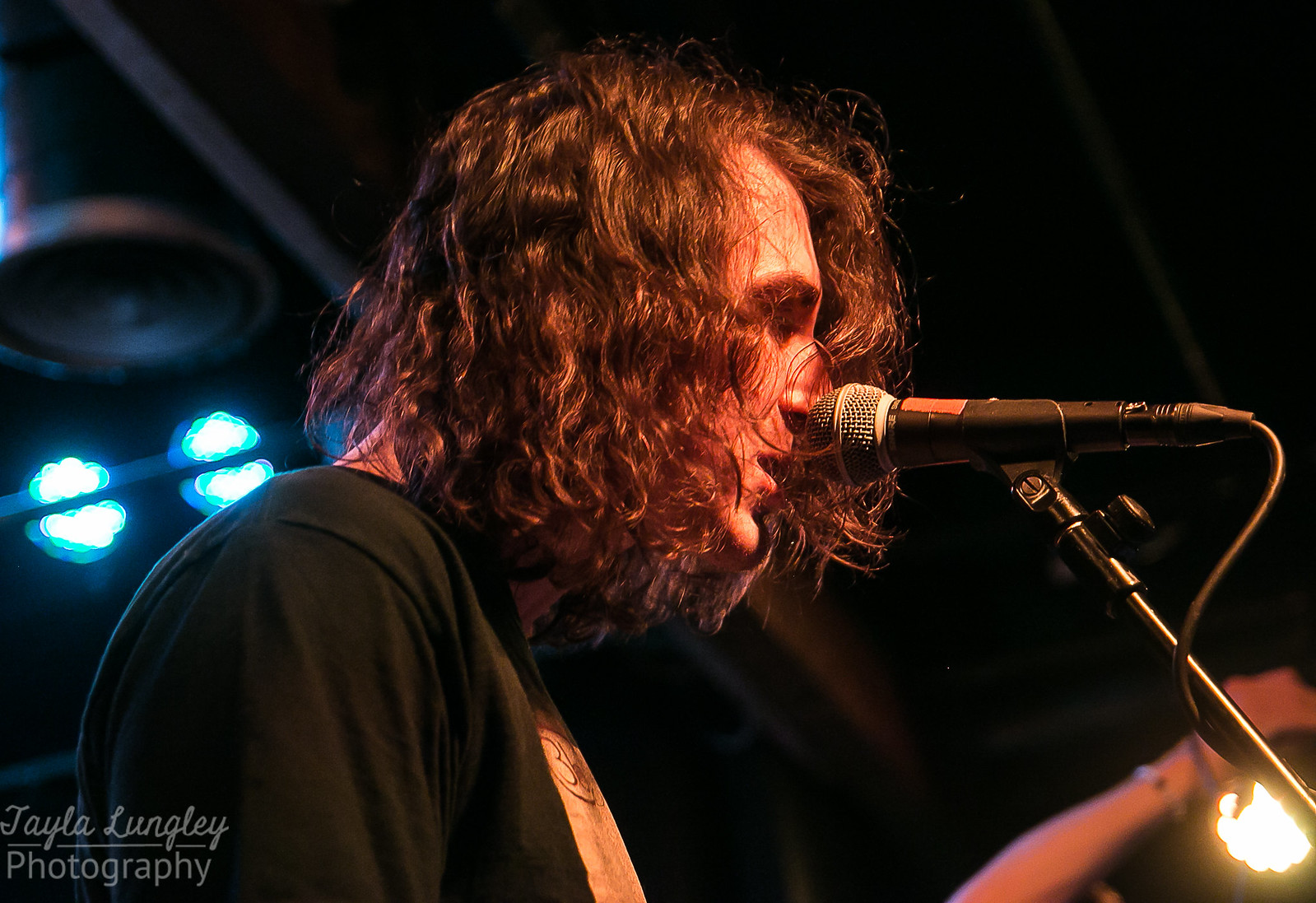The photograph captures a young male singer with long, messy brown hair that falls to his shoulders, partially covering his face. He is facing towards the right and singing into a sleek black microphone with a silver ball on the end, which is positioned close enough to nearly obscure his nose. The microphone features a small amber-colored square on top, and its wire descends and veers to the left before disappearing from view. The singer is dressed in a black shirt and has a light orange strap with black writing draped over his shoulder, hinting that he might be playing a guitar, though the instrument itself is not visible in the photo. 

The setting is dimly lit with a predominantly black background, punctuated by four teal-colored lights shining through on the left side and a bright yellow light illuminating the bottom right corner, reflecting off the microphone stand. A person's hand is also visible in the lower right, suggesting the presence of other performers on stage. The lower left corner of the image features the text "Tayla Lungley Photography" in gray, noting the photographer's credit. 

The overall atmosphere is that of a professional live performance, with focused lighting adding to the scene's dramatic and immersive quality.